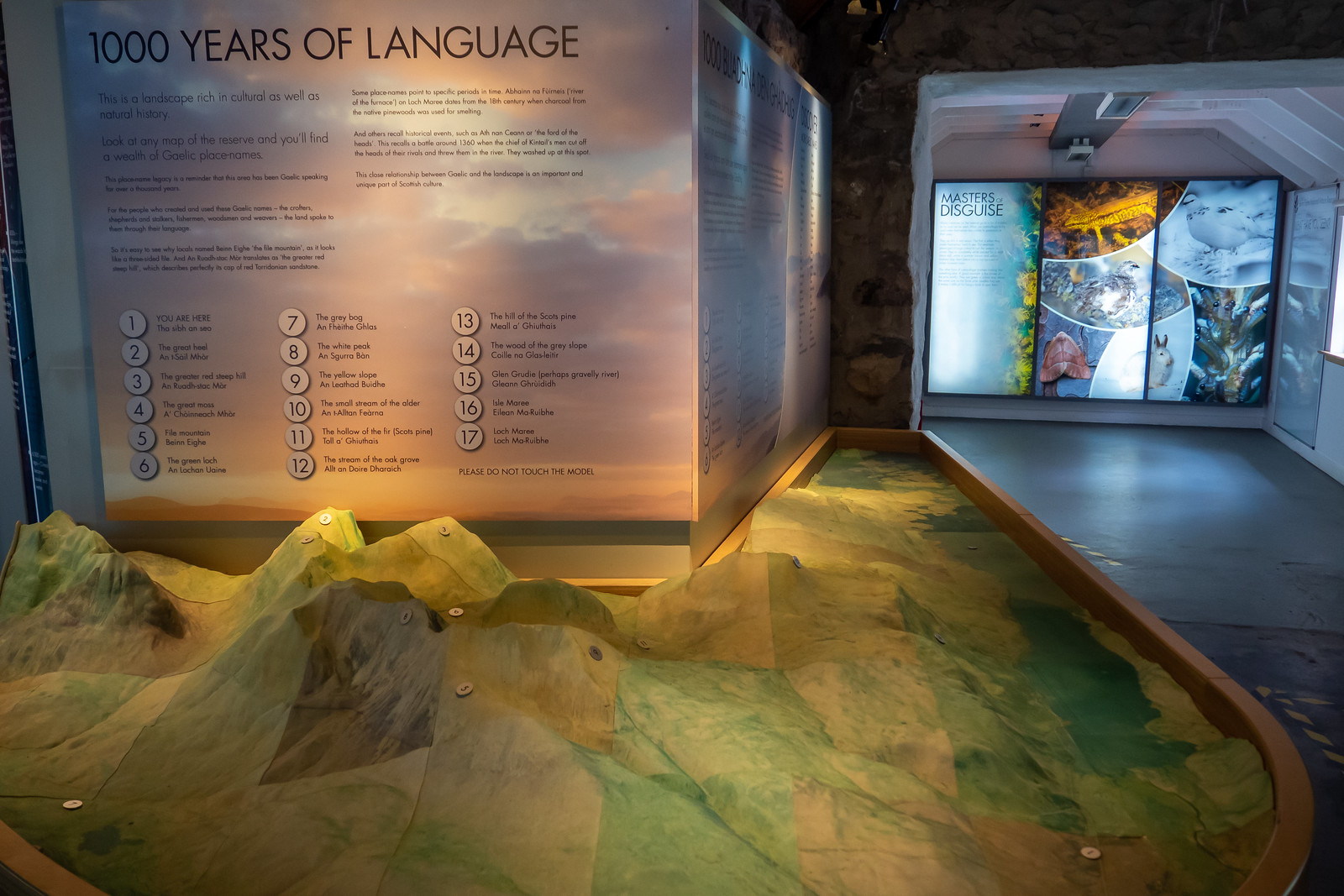This detailed image depicts the interior of a museum featuring multiple exhibits. The ground surface appears to be made of hard concrete. Prominently, in the bottom left corner, there's a detailed topographical model of a mountain rendered in shades of green, light green, blue, tan, and beige. This model is adorned with white circles, each numbered from 1 to 17, which correspond to black text descriptions.

Along the purple L-shaped wall in the top left, large black letters spell out "1,000 years of language," accompanied by several paragraphs of text that are difficult to read due to their small size. To the right of the mountain model, a gray walkway leads to a hallway illuminated with colorful screens displaying vivid images of plants or animals. These screens, captioned with "Masters of Disguise" in the upper left corner, add a dynamic element to the indoor setting. The ensemble of exhibits, dominated by shades of gray, brown, purple, pink, light blue, orange, and yellow, immerses visitors in an informative and visually captivating museum environment.